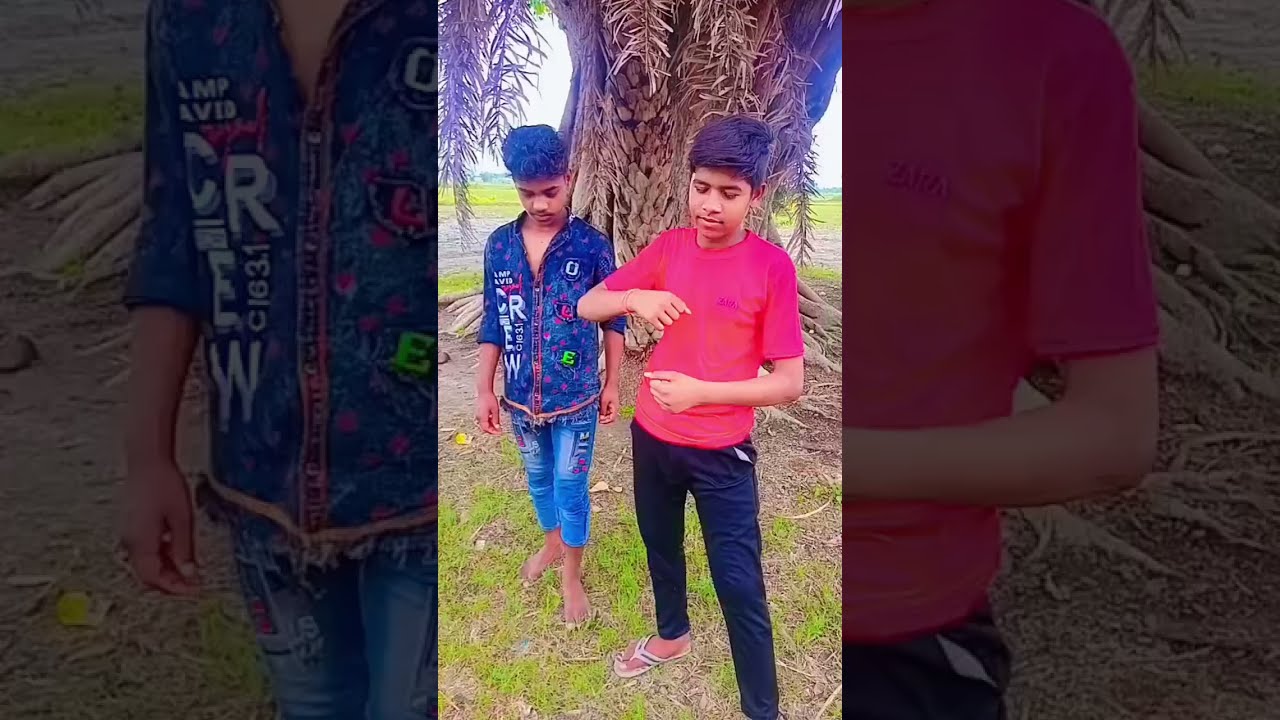This image captures two early teenage boys standing in front of a large tree with broad fronds on a bright day, possibly in a tropical setting like the Philippines. The central vertical strip of the photograph is clear, while the left and right side panels are darkened and amplify portions of the main image. 

The boy on the right foreground wears a red t-shirt, dark blue pants, and white flip-flops. He is intently looking at an indistinct object clinging to his right hand. His arms are extended in front of his torso, with one hand on top of the other. The boy behind him to the left wears a blue patterned button-down shirt and blue jeans, and he is barefoot. He is looking downwards, seemingly not engaged in any particular activity. Both have short to medium-length dark hair. 

The boys stand on a grassy field with a possible road curving around the tree in the background. The sky is bright, illuminating their natural surroundings, which adds to the overall vibrant, tropical atmosphere of the scene.